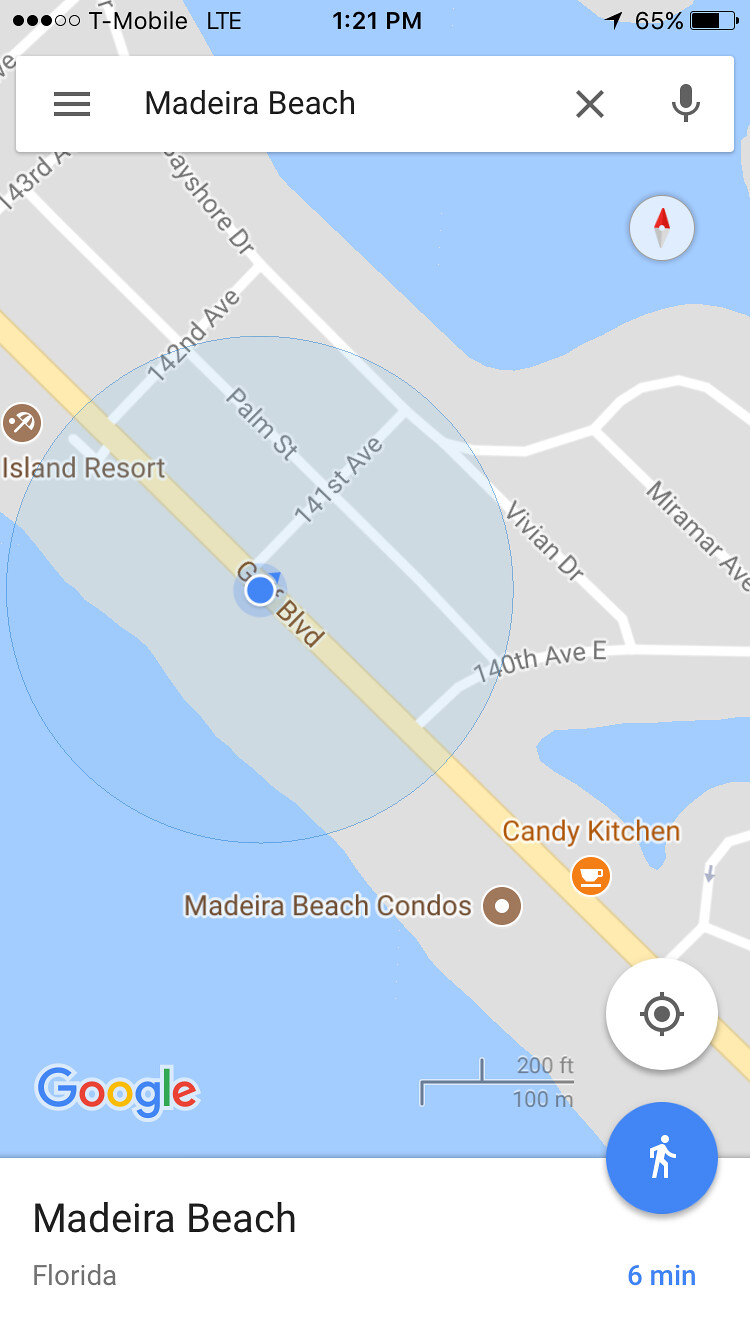This image is a detailed screenshot of a Google Maps application on a smartphone, displaying the area around Madeira Beach, Florida. The phone is connected to T-Mobile's LTE network, with the signal strength, time (1:21 p.m.), and battery level (65%) visible at the top. The GPS screen prominently features Madeira Beach in a white search bar at the top and a blue dot indicating the user's location on a boulevard. Surrounding streets such as 142nd Avenue, Palm Street, Vivian Drive, and Miramar Avenue are visible. Notable landmarks include Madeira Beach Condos, Candy Kitchen, and Island Resort. The map shows the coastal layout of Madeira Beach with water bodies on either side, and the bottom of the screen notes a walking distance to Madeira Beach, Florida, represented by a blue walking person icon, estimated at six minutes. Google’s logo is positioned at the lower left corner of the screen.